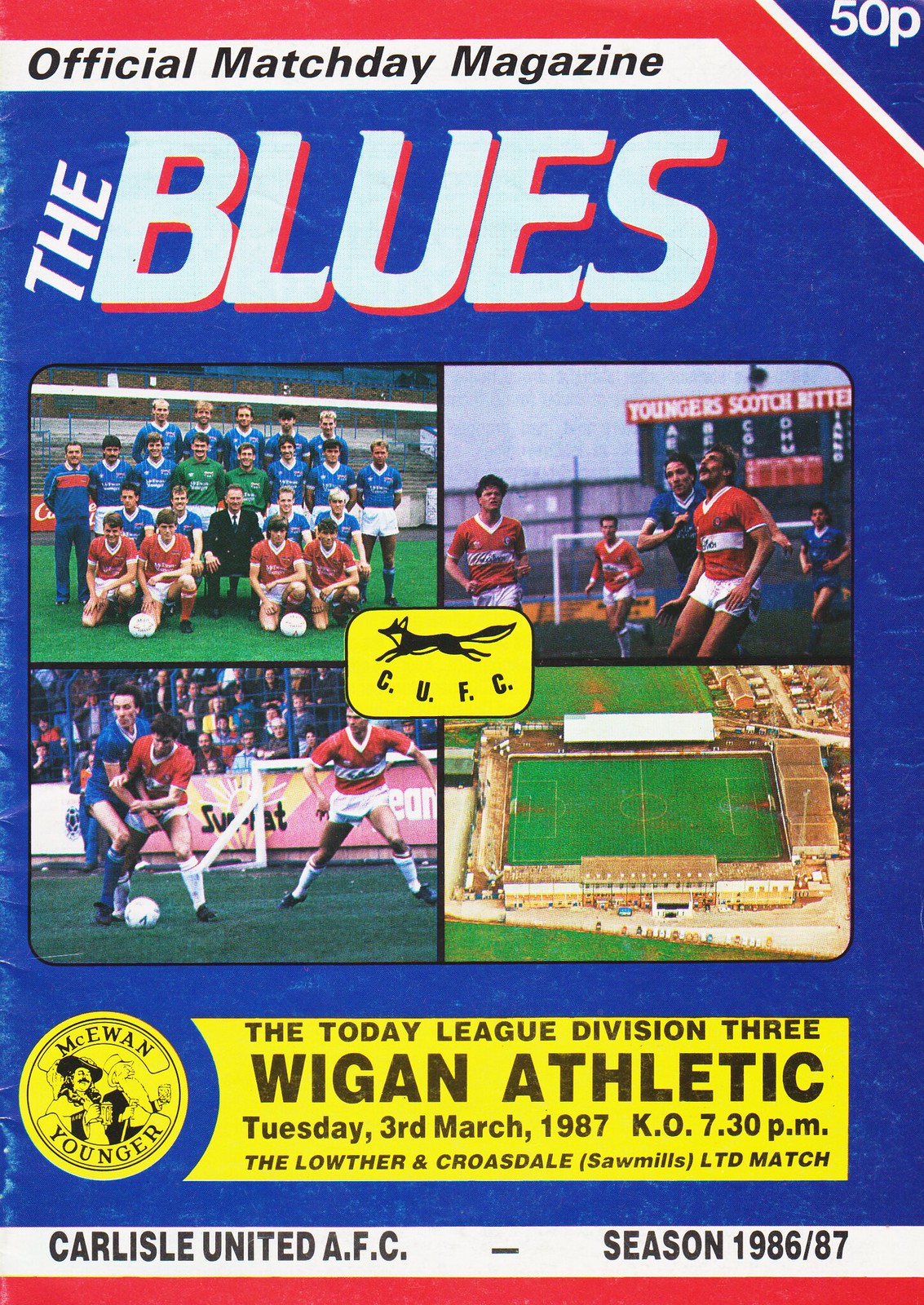The cover of this vintage soccer magazine, titled "The Blues," features a predominantly blue, red, white, and yellow color scheme with a price tag of 50p in the top right corner. At the top, the magazine is labeled "Official Match Day Magazine." The main section consists of a 2x2 grid of four photographs. The top left photo is a team picture, with players gathered in front of a net and the manager or owner positioned centrally. The top right photo captures an action shot of teams in red and blue competing on the field. The bottom left image also showcases a soccer match between red and blue teams. The bottom right photograph provides a bird's eye view of the soccer stadium. Central to these images is the acronym C-U-F-C, accompanied by a fox. Below the photographs, a yellow text box reads: "The Today League Division III, Wigan Athletic, Tuesday, 3rd March 1987, K-O 7.30 p.m." Additionally, there's a mention of "The Lother and Crosedale Sawmills LTD Match" at the bottom.